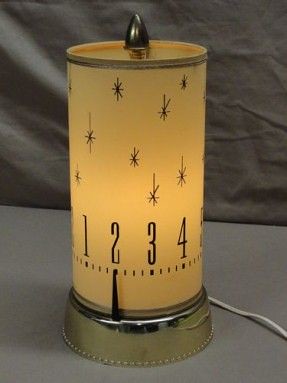A close-up image of an electric light housed within a cylindrical canister, emitting a warm, candle-like glow in a pale yellow-orange hue. The canister is decorated with small, black star illustrations and features the numbers 1 to 5, in black, arrayed in a circular sequence around its lower portion. Below these numbers is a gauge, with a pointer currently indicating the number 2. The canister rests atop a gold-colored base from which a white electric cord extends out from the bottom right. The entire setup is framed against a plain gray background, accentuating the light’s warm and cozy ambiance.